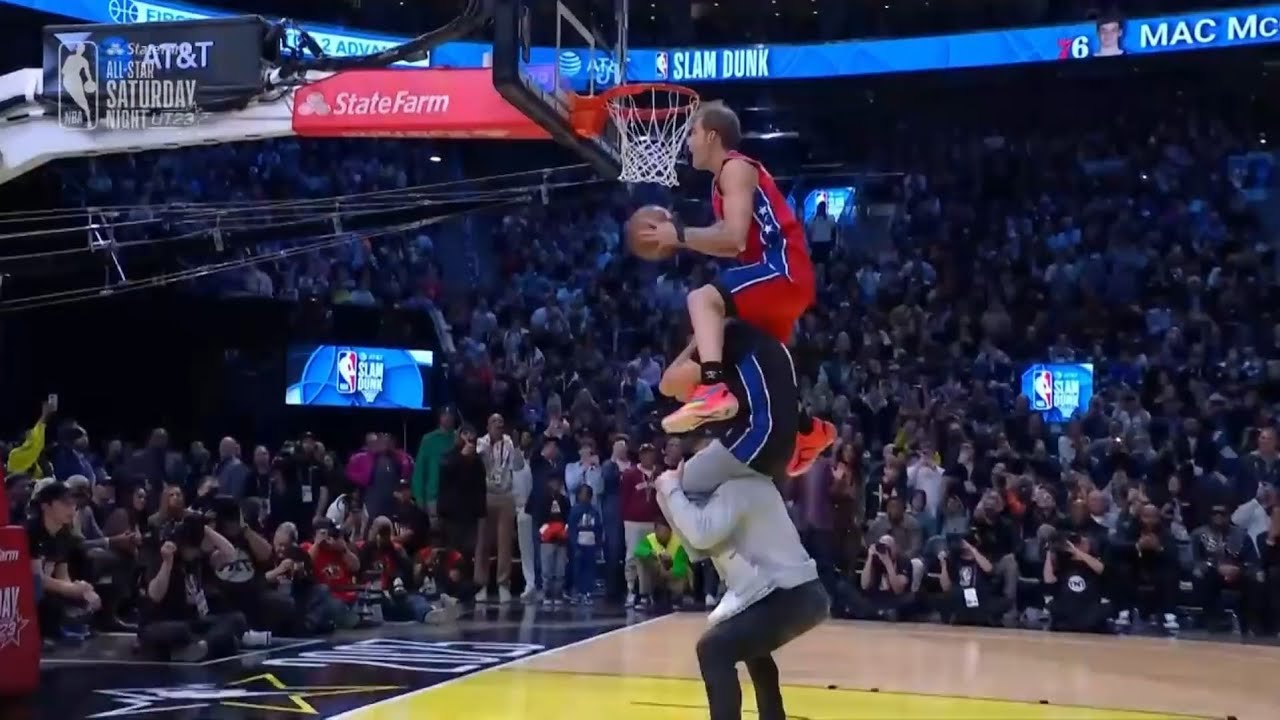The image depicts a vibrant basketball game during a halftime show, highlighted by a staggering feat of athleticism. Three individuals are stacked on top of one another in the center of the court: the bottom man wears black pants and a gray shirt, the middle man sports a black and royal blue uniform, and the topmost man dons a red uniform with blue stripes, red shorts, pink and white sneakers, and black socks with decorations. The top man is grasping a basketball just below the net, seemingly preparing for an impressive dunk. The crowd, which forms a large, attentive backdrop, watches intently. The court beneath them is yellow and tan, framed by a blue banner overhead, displaying partial text such as "MAC" and "slam dunk.” Further context is provided by advertisements like AT&T's "All-Star Saturday Night" and State Farm. TVs in the background add to the lively atmosphere, capturing the thrilling moment.